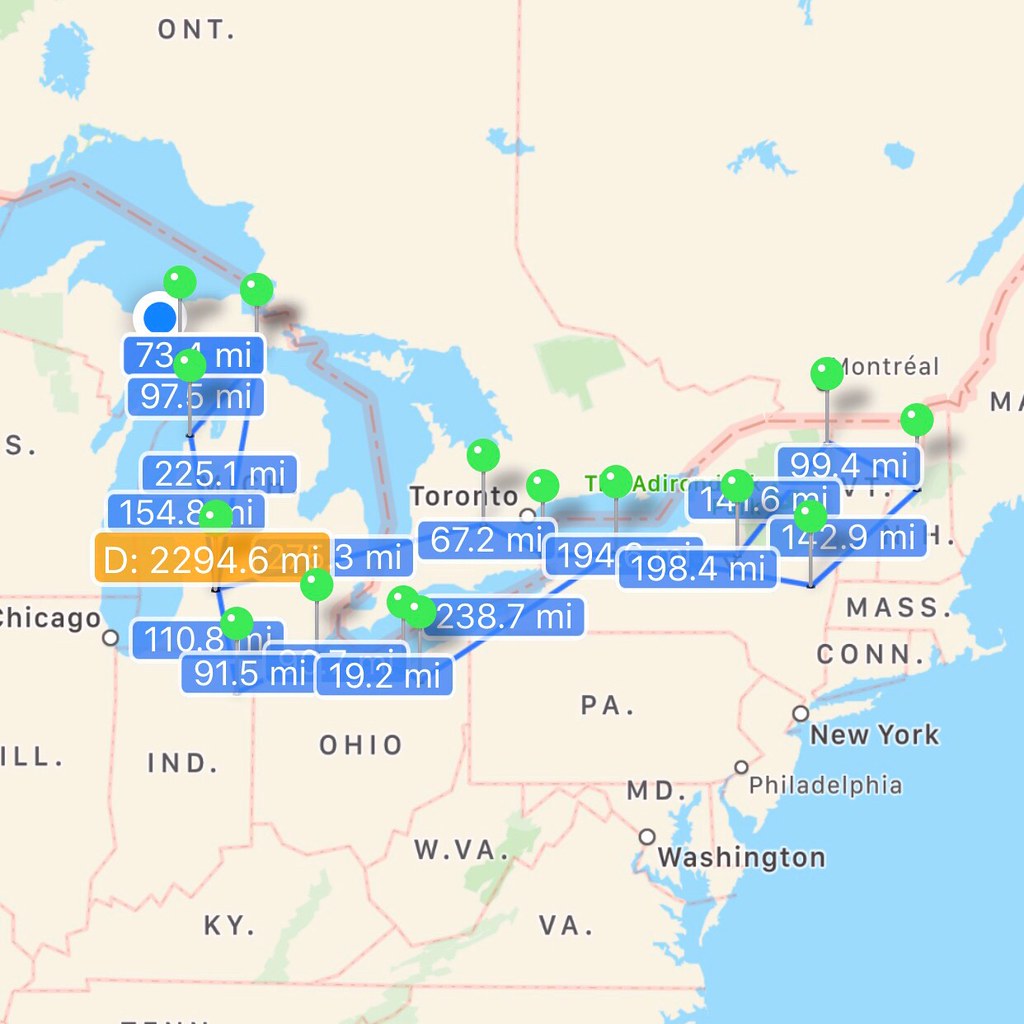A detailed photo features an intricate network of pins and strings mapping out connections between various major cities globally. Though the cities are not labeled, the dense web of lines crisscrossing the image vividly depicts the complex relationships and routes linking these urban hubs. Each pin represents a city, carefully placed to illustrate its geographical location relative to the others. The strings connecting these points create a visually striking illustration of global interconnectivity, highlighting the extensive and intertwined nature of international networks.